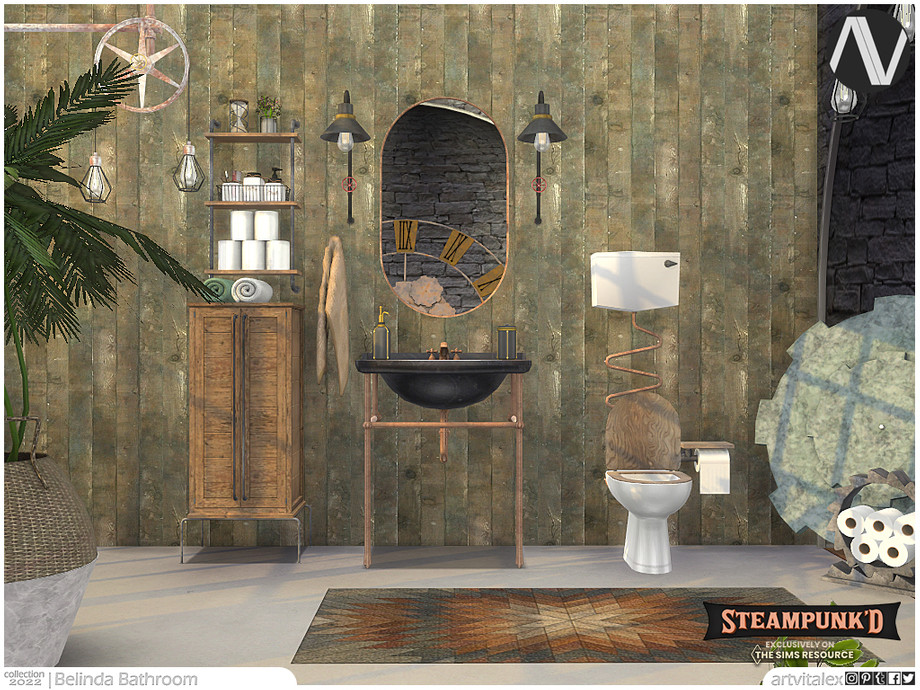The image is a detailed, computer-rendered depiction of a steampunk-themed bathroom, described in various segments with subtle differences. At the bottom right corner, it includes the label "Steampunked exclusively on The Sims Resource, Art Vitalex," along with logos for Pinterest, Facebook, and Twitter. Additionally, the words “Collection 2022, Belinda Bathroom” appear on the left.

The bathroom features a color palette predominantly of browns, complemented by greens and grays. The back wall is covered in either strips of brown wallpaper or tile. Centered in the scene is a stylish black pedestal sink, shaped like a bowl, equipped with a faucet. Mounted above the sink is an oval mirror flanked by lights with black tin shades. To the left of the vanity stands a wooden stand with open shelves stocked with toilet paper, toiletries like lotions, soap, a toothbrush, and a green and white rolled-up towel. Hanging from a pulley system are Edison lights, enhancing the steampunk aesthetic.

Adding to the rustic charm, on the left side of the scene is a large basket with a plant growing in it. The bathroom floor is gray, and a rug in shades of gold, tan, and black lies in front of the sink. More details reveal a white porcelain toilet with a wooden seat and backrest. A copper pipe connects the toilet to a wall-mounted water tank. There is also an ornate mirror reflecting part of a wall clock with Roman numerals. A wooden holder with toilet paper stands to the right of the toilet, next to a large metal blade adding to the industrial vibe of the bathroom. The elements and meticulous details combine to create a striking, steampunk-inspired bathroom within The Sims universe.